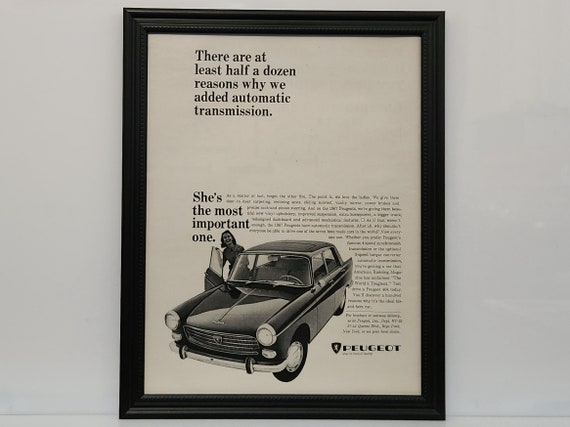The image depicts a vintage black-and-white advertisement for Peugeot, framed and possibly hung on a slate grey wall. The frame is black and rectangular, resembling a plaque. The main focus of the advertisement is a 1960s Peugeot car with emphasis on its new automatic transmission feature. The top portion of the ad contains significant negative space with the text: "There are at least half a dozen reasons why we added automatic transmission. She's the most important one." Below this text, a woman is captured laughing as she stands by the open passenger door of the car, facing the camera with her right hand holding the door. Positioned to the right of the car image is the Peugeot name accompanied by a logo. The entire ad conveys a somewhat dated message highlighting the convenience or safety of the automatic transmission, likely suggesting it makes the car easier for women to drive. The overall setting suggests it may be a product photo inviting customers to order this reproduction print.